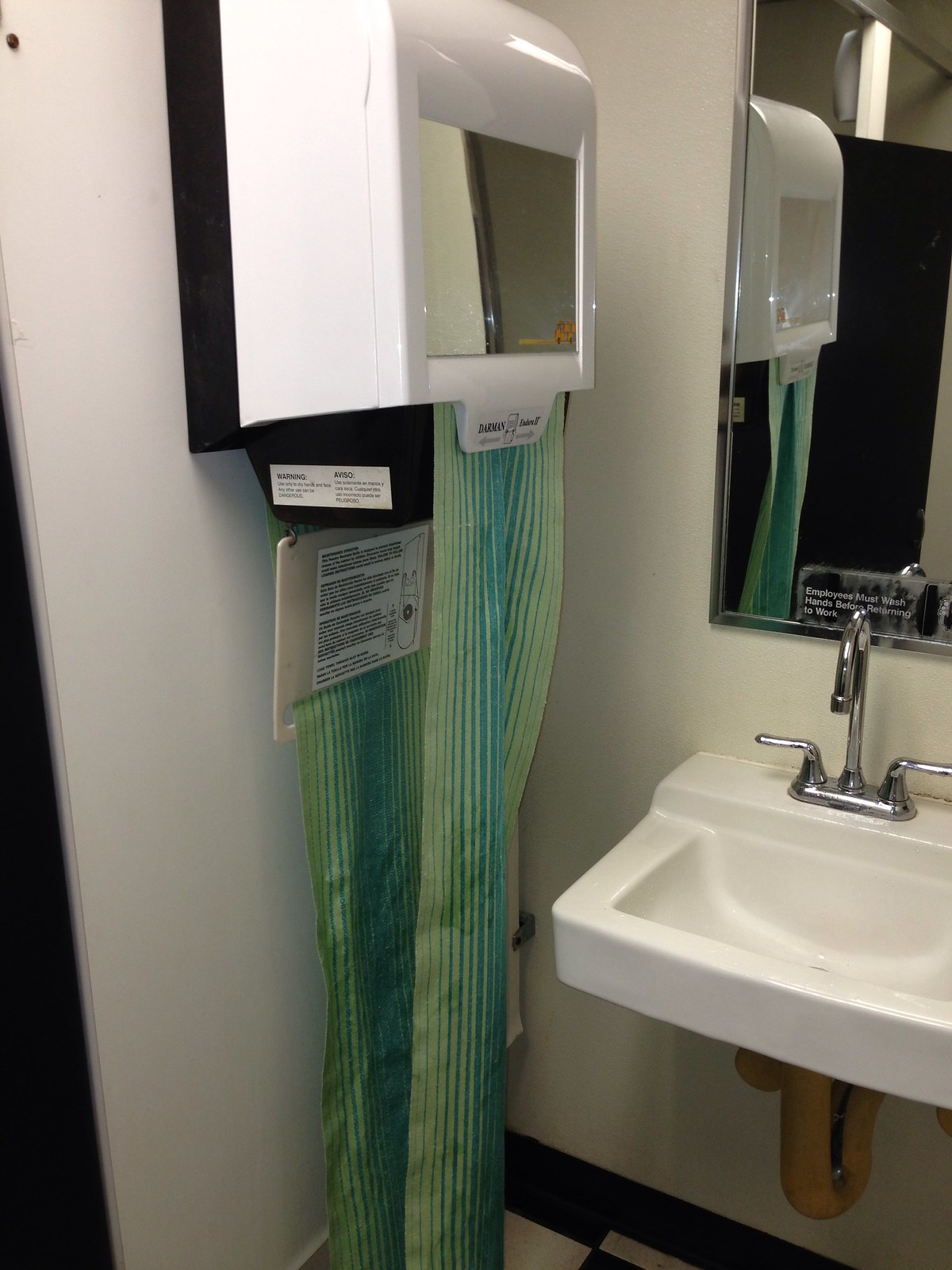The image is taken inside a public restroom with a white and black tile floor. Prominently featured is a single white hand-washing sink with a silver chrome faucet and two metal knobs for hot and cold water. Beneath the sink, there is an off-white pipe that appears to be deteriorating. Above the sink, a vertical rectangular mirror with a metal frame is mounted on the wall. A small, unreadable sign is attached at the bottom of this mirror. 

To the right of the sink, there is an old-fashioned towel dispenser attached to the white wall. This dispenser is rectangular with black trim and has a smaller mirror cut into its front. Below the mirror on the dispenser, there is a large instruction sign. The towel hanging from the dispenser is a continuous loop of cloth in varying shades of green and blue, overextended and touching the tile floor.